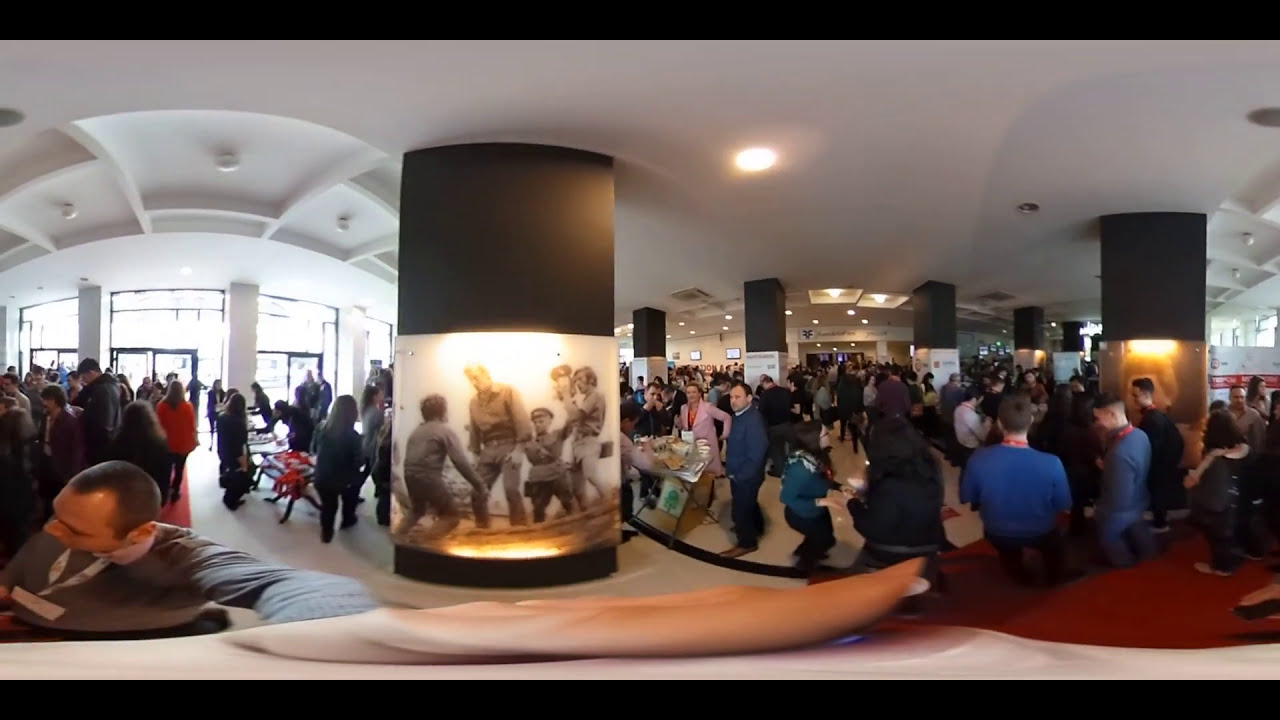The image depicts a crowded indoor setting, possibly a museum or an art gallery, bathed in natural daylight from windows and glass doors. The expansive room has white ceilings with deep inset lights and numerous black pillars adorned with historical black-and-white images. Dominating the center is a gray column featuring a wartime photograph, possibly from World War II, showing soldiers and an old-style camera. The crowd, over fifty people, is densely packed, mingling, talking, and observing various displays. A noticeable individual in the lower left corner, likely the photographer, is a Caucasian male with a white lanyard and name tag, wearing a long-sleeved gray shirt. The panorama effect used in the photograph distorts some lines, curving straight edges and expanding certain areas, adding an interesting visual twist to the busy, informative atmosphere of the room.